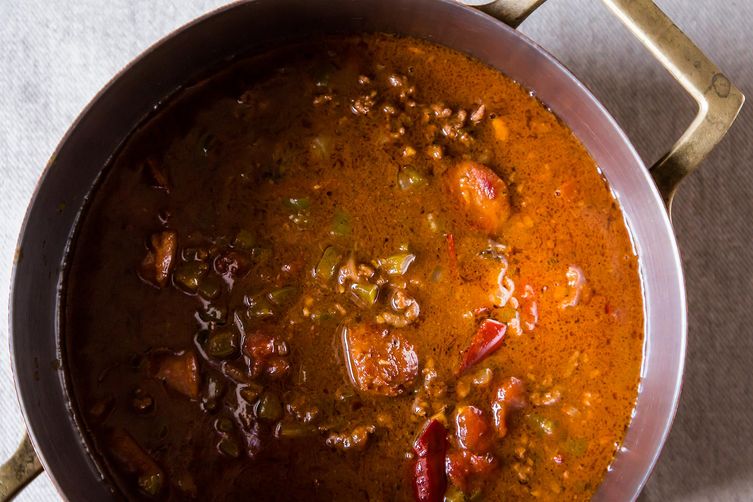The image depicts a large, stainless steel pot, distinguished by its copper-colored handles, one of which is visible in the upper right corner, with another partially visible at the bottom left. The pot rests on a light-colored fabric or surface, which could be whitish gray or light blue. Inside, the pot contains a reddish-brown broth that resembles chili or stew. The contents include recognizable chunks of ground beef, kidney beans, slices of sausage, diced green vegetables, red chili peppers, red bell peppers, and potatoes. Additionally, there are some unidentifiable miscellaneous lumps that could be pieces of either meat or tofu. The visible ingredients are complemented by seasoning and bits of rice dispersed throughout the broth. The mixture is not actively boiling; it is simply resting in the pot, showcasing a rich, hearty, and complex stew or chili.